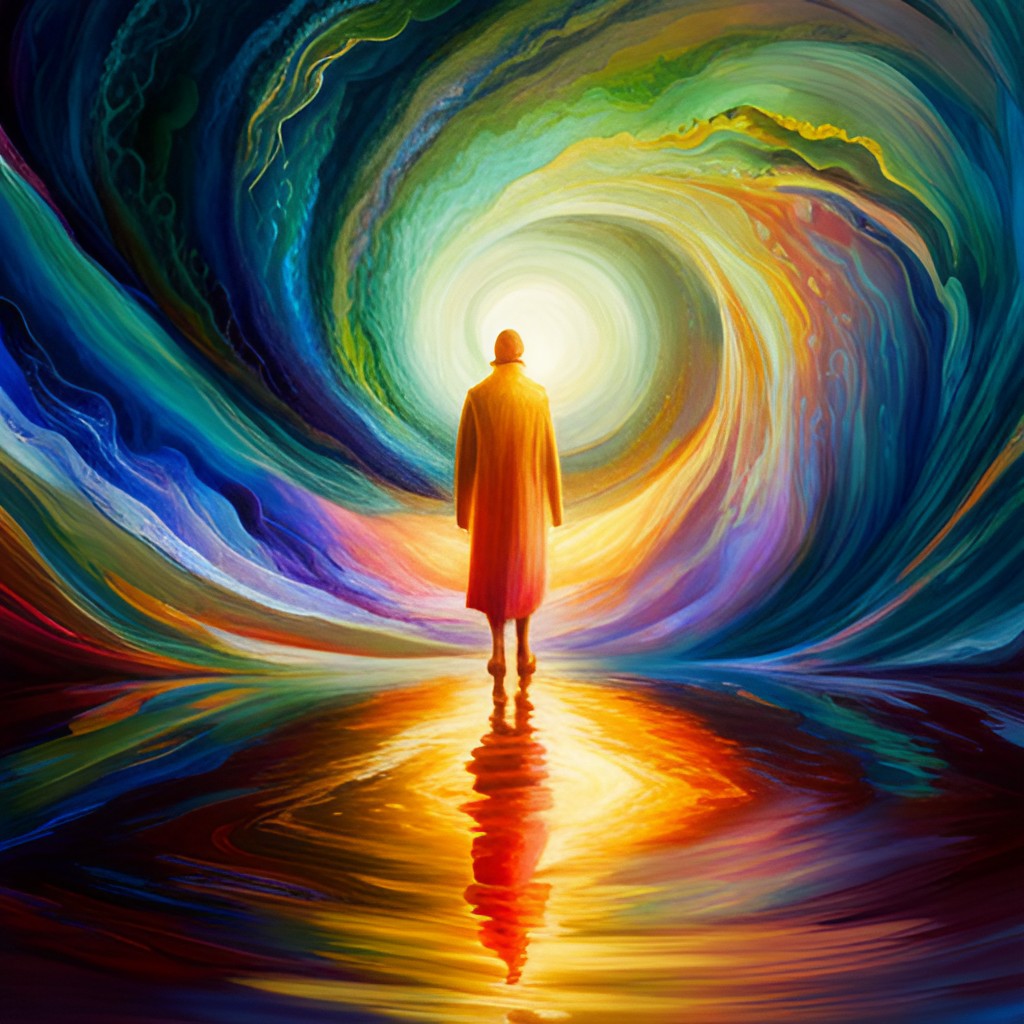In this vibrant and dreamy square painting, a lone figure, possibly female, stands at the center. The figure is depicted from the back, adorned in a long, richly colored coat that flows just past the knees. The coat features a dynamic palette of oranges, yellows, and pinks, adding warmth to the image. On their head, the figure wears a brimmed hat, complementing the colorful ensemble. They appear to be walking on a rippling, reflective surface, reminiscent of water, which captures a distorted but mesmerizing mirror image of the figure and their surroundings.

Surrounding the figure is a captivating blend of swirling colors, forming a tunnel-like structure that they seem to be walking towards. This spiral pattern starts from a central white or whitish-yellow core and radiates outwards through an evolving spectrum of blues, greens, reds, purples, and oranges. The swirling colors give the illusion of depth and motion, resembling a twilight zone-like vortex. The reflection beneath the figure further enhances the sense of dreamlike tranquility and endless continuity, mirroring the vivid, swirling patterns above. The entire scene is both surreal and immersive, inviting viewers into a world of color and light.